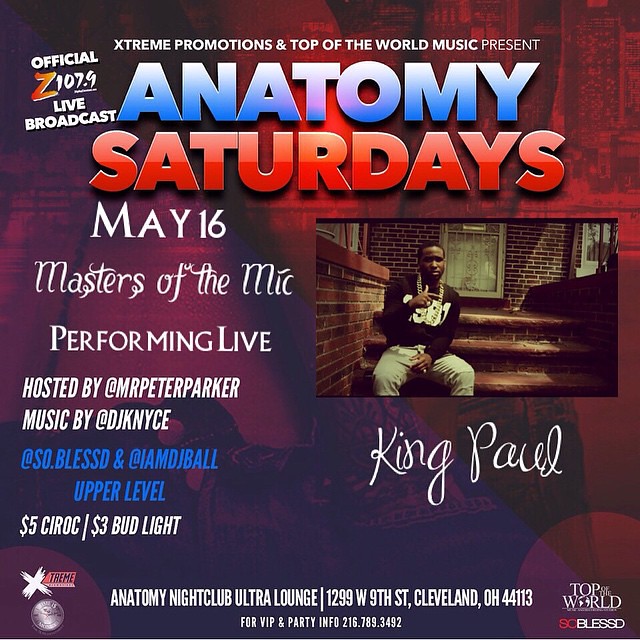The image is an informational poster for an event. At the very top, in all-caps white font, it reads "Extreme Promotions and Top of the World Music Present." Beneath this, in large blue font, the word "Anatomy" appears, followed by "Saturdays" in red font. Further down in white font, it states, "May 16th, Masters of the Mic Performing Live," hosted by "@MrPeterParker" and featuring music by "@DJKNYCE," "@SoBlessed," and "@IMDJBellUpperLevel." The event offers $5 Ciroc and $3 Bud Light. 

A central feature of the poster is a picture of a black man, presumed to be one of the DJs or performers, sitting on steps. He is wearing jeans, a black sweater with white writing, and several gold chains. Underneath this picture, "King Paul" is written in cursive. The background of the poster is mostly red with some indistinct elements. At the bottom, it mentions that the event takes place at Anatomy Nightclub Ultra Lounge on 9th Street, Cleveland, Ohio, and includes contact information.